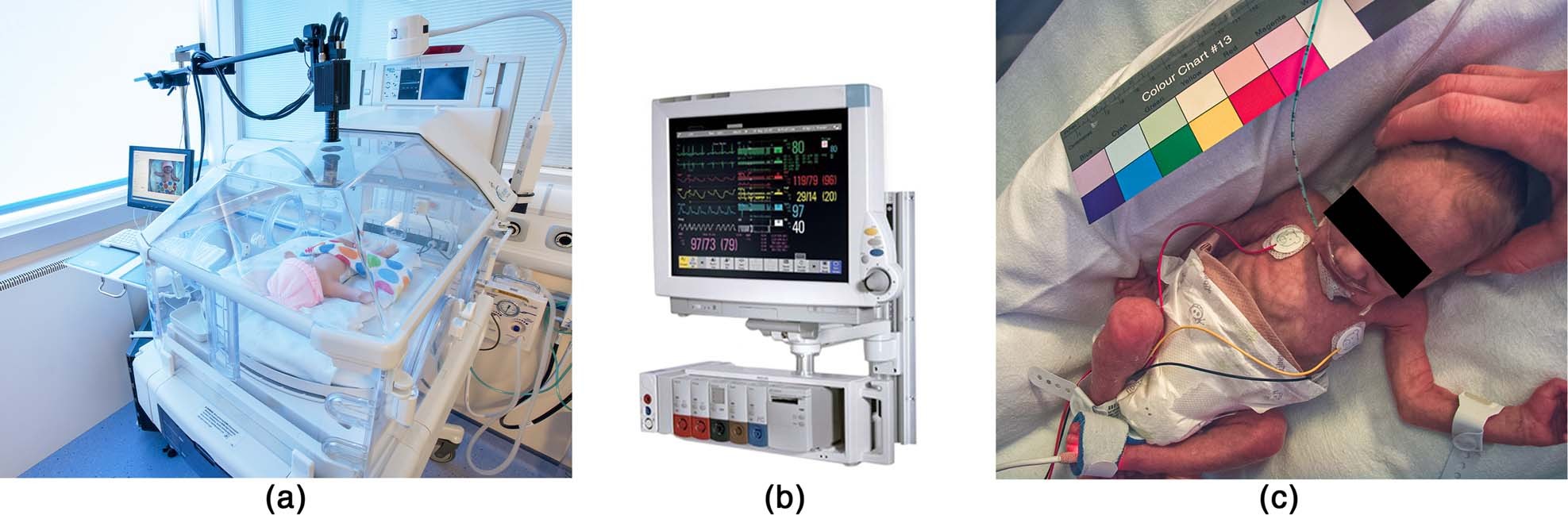The provided images depict various aspects of a neonatal unit at a hospital. The first image (A) features a baby lying in an incubator, swaddled with a polka dot blanket and wearing a pink hat. The incubator is surrounded by advanced medical equipment, emphasizing the critical care environment. The second image (B) displays a hospital monitor against a white background, with various readings such as heartbeat and blood pressure, and buttons of different colors at the bottom. The third image (C) shows another baby, positioned at an angle, with a black bar obscuring its eyes. The baby, dressed only in a disproportionately large diaper, is connected to several monitors and appears quite fragile. Beside the baby, there is a color chart labeled "Color Chart #13," featuring a range of colors from purples to whites. Additionally, a hand is gently placed on the baby's head, suggesting care and monitoring. Each image is labeled respectively with lowercase letters in parentheses: (a), (b), and (c).